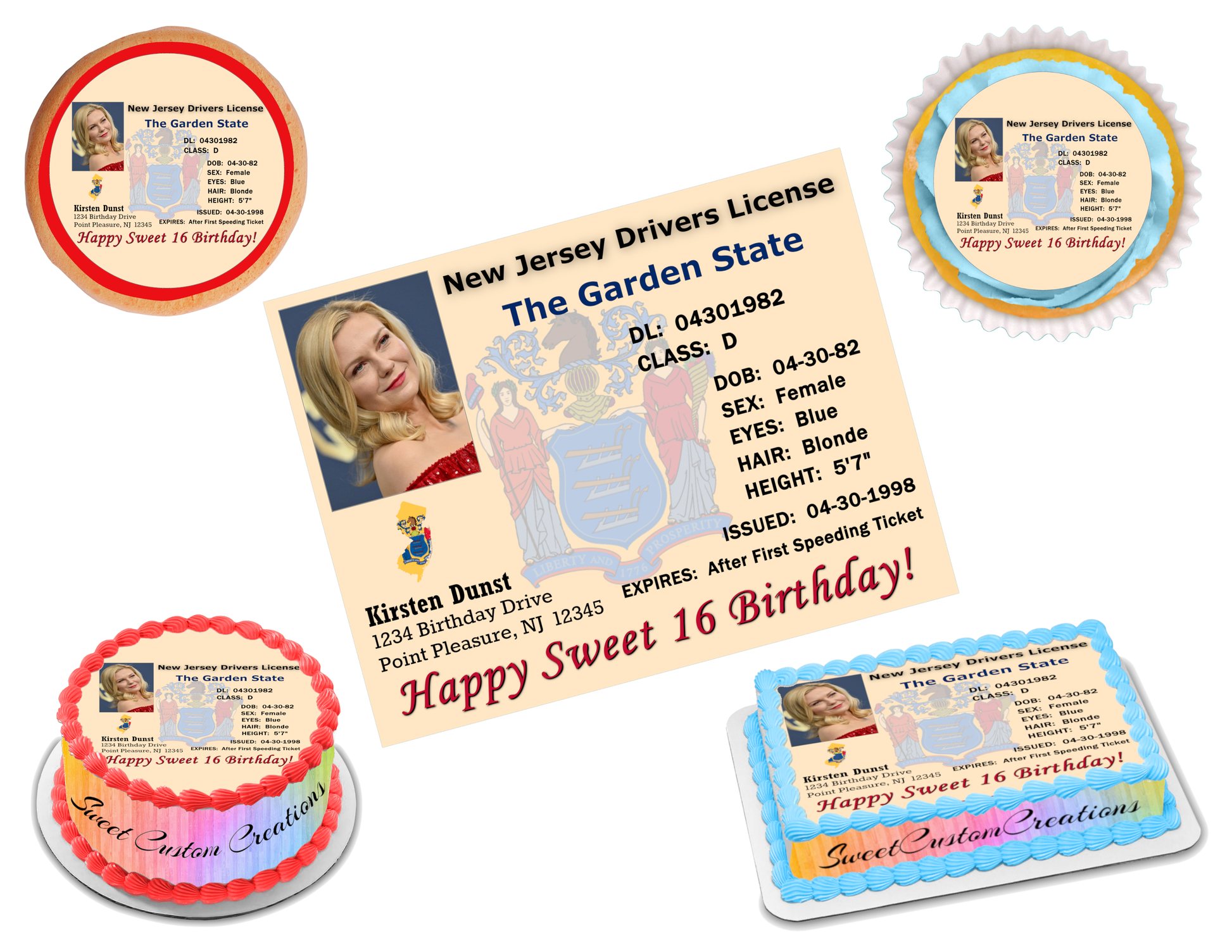This image showcases a collection of personalized Sweet 16 birthday items set against a white background. Central to the image is a beige-colored mock-up of a New Jersey driver's license, whimsically featuring actress Kirsten Dunst's photograph and personal details such as height and sex. The license displays "Happy Sweet 16th Birthday," and humorously notes, "Expires after first speeding ticket." Surrounding the mock driver's license are four cakes, each featuring the same license image printed on their surface. The cakes include a round one with red icing, a rectangular one with blue icing labeled "Sweet Custom Creations," implying the name of the business, and additional circular and rectangular cakes. The corner also reveals a possible prize ribbon and a saran-wrapped cookie, both adorned with the driver's license mock-up design. The entire collection forms a playful and customized birthday party set-up.